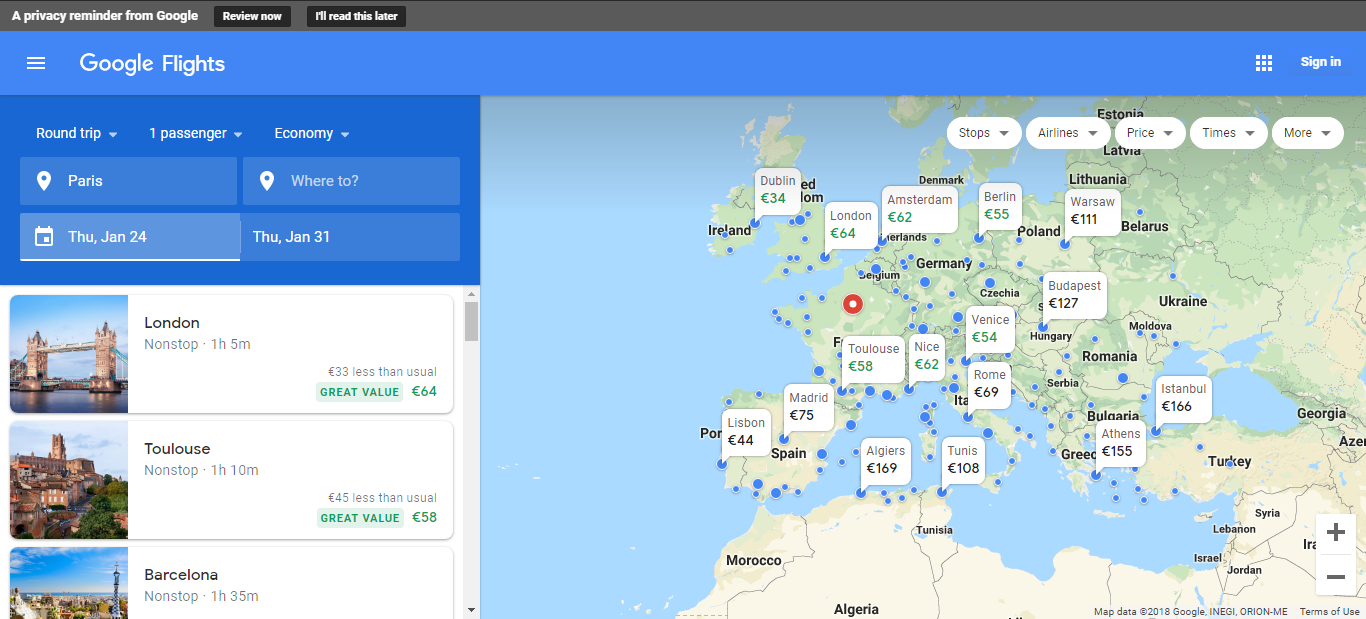The image displays a screenshot of a website interface, possibly viewed on a desktop or tablet, given its wider-than-tall aspect ratio, approximately 2.5 times wider. The header of the page features a gray bar spanning the entire width, occupying around 5-10% of the vertical space. In the upper-left corner of this gray bar, white text reads "A privacy reminder from Google," accompanied by two black buttons with white text: "Review now" and "I'll read this later."

Beneath the gray bar, a light blue navigation bar stretches horizontally across the width of the page, estimated to take up about 15% of the image's height. On the left side of this bar, three horizontal white lines represent a menu icon next to the text "Google Flights." On the right end, there is a 3x3 grid icon followed by the text "Sign in."

Below the light blue bar, the main interface of Google Flights becomes visible. Towards the top-left, the user has selected flight preferences: "Round trip," "1 passenger," and "Economy." The departure and destination details show that the origin is Paris, with the destination field still blank, indicated by the placeholder text "Where to." The travel dates are set for Thursday, January 24th (departure) to Thursday, January 31st (return).

The left section of the interface features options for selecting flight details, while the right section displays a map of Europe. Moreover, below the flight options, there are three suggested travel locations to choose from. The layout and design suggest a user-friendly interface aimed at streamlining the flight booking process.